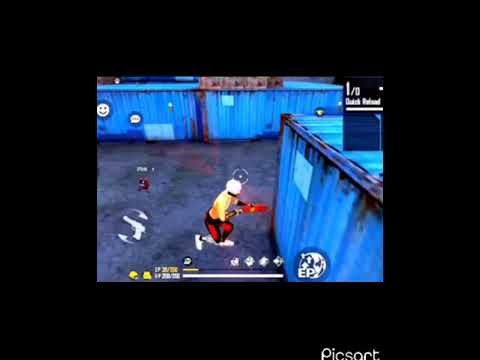The image is a still shot of a video game screen featuring an action scene from a shooter game. Central to the picture is a cartoon-style character wearing red pants, a yellow shirt, and a primitive white helmet. The character is crouched in an action stance, holding a weapon with red accents, and appears ready to shoot. The character is positioned on a gravel or cement ground, partially hiding behind a large blue shipping container that shows signs of rust and grime. To the right and behind the character are additional blue shipping containers, similarly weathered. In the lower portion of the screen, two horizontal bars suggestive of health or energy stats can be seen, as well as a score stats bar with numbers. The character is also targeted by a gun scope indicated by a white dot with a circle around it on their head. The entire image is framed by a complete black border, giving it a cinematic feel.